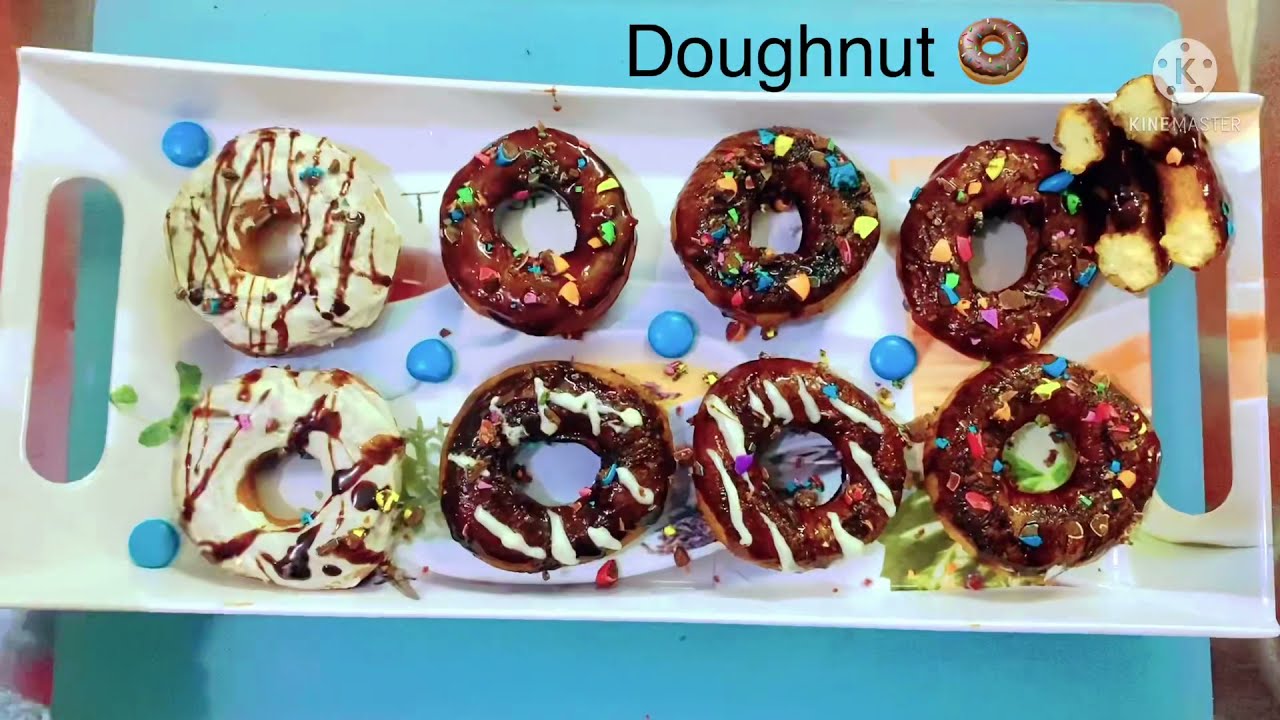This full-colored promotional photograph, set against a blue background, depicts an enticing variety of donuts arranged on a long white serving tray with concave edges and handles on both sides. Eight whole donuts and one half-donut are neatly placed in two rows of four each, topped with diverse and colorful decorations. Some donuts are chocolate-covered with vibrant sprinkles or broken M&Ms, while others are glazed white with chocolate or caramel drizzle. Blue chocolate candies are thoughtfully scattered around the donuts, enhancing the visual appeal. At the top of the image, the word "donut" is prominently displayed beside an image of a frosted donut. In the top right corner, a white circle with five hole punches encloses the letter 'K', a logo symbolizing KineMaster. This image is sure to make you hungry and showcases the delightful assortment of donuts in a meticulously arranged setup.